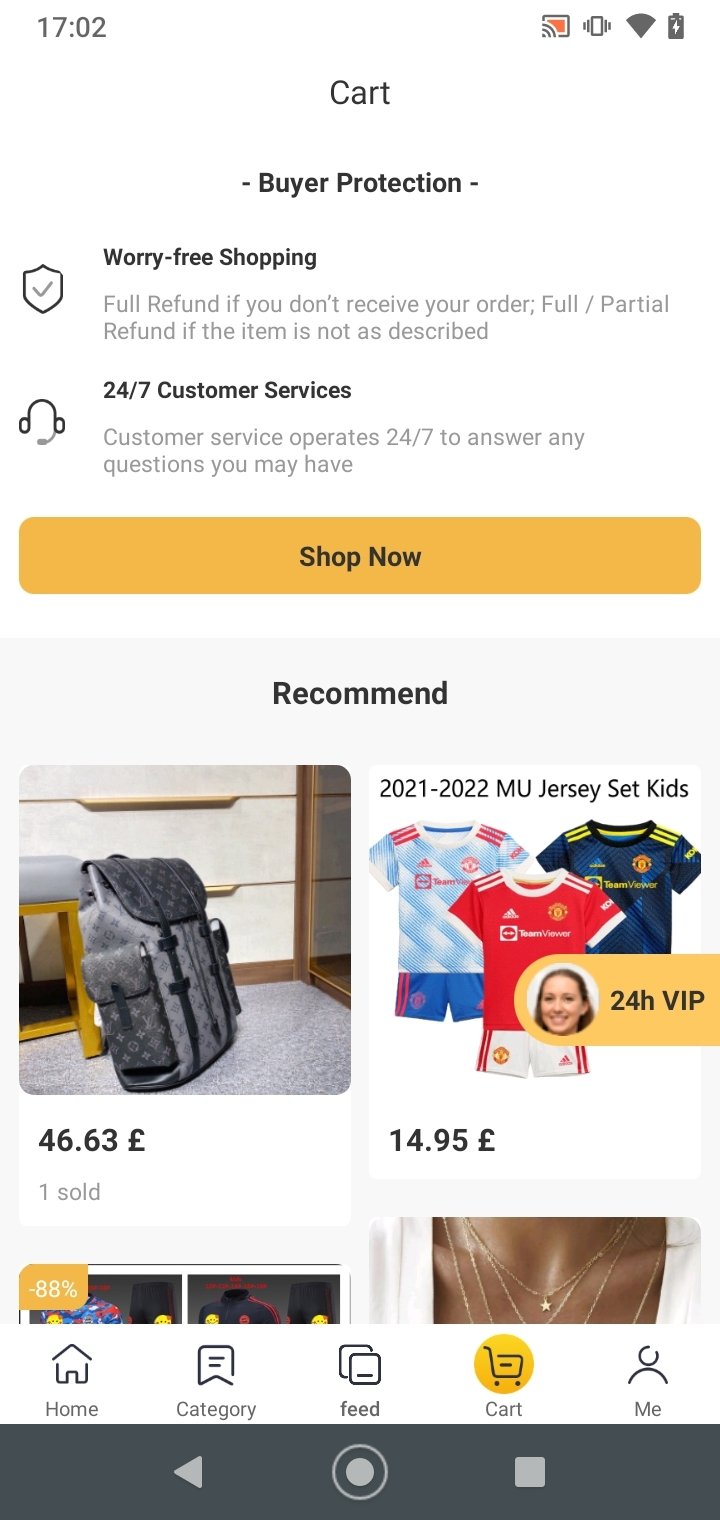A mobile screenshot of a shopping website displays a typical user interface with essential features and promotions. At the very top left corner, the military time reads "1702", while the top right corner showcases four symbols, including a battery icon. Centered at the top is the word "Cart."

Just below this header, a section titled "Buyer Protection" emphasizes "Worry-free shopping" with guarantees: "Full refund if you don't receive your order" and "Full/partial refund if the item is not as described." A shield symbol with a checkmark accompanies this text.

Further down, "24/7 Customer Services" is highlighted, showing that customer service operates around the clock to assist with inquiries. This is paired with a headset icon. A prominent yellow button labeled "Shop Now" stretches across the width of the screen.

Underneath, the section "Recommend" features product recommendations displayed in a grid. The first row, fully visible, includes a gray backpack on the left and three sets of boys' clothes (each set comprising a shirt and shorts) on the right. The boys' clothes section includes a headshot labeled "24HVIP." Partially visible on the next row, the right item appears to showcase women's necklaces displayed on models' necks.

At the bottom of the screen, navigation icons are labeled "Home," "Category," "Feed," "Cart," and "Me," each with corresponding icons above the text.